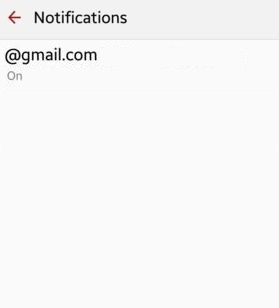The image depicts a horizontally-oriented, light gray rectangular interface with a slightly darker light gray strip running across the top. On this strip, there is a prominent red arrow pointing to the left, accompanied by the word "Notifications" in black text. Below this strip, on the lighter gray background, is the text "at gmail.com" in black, left-justified. Beneath it, in an even lighter gray text, is the word "on." The overall color scheme of the interface includes shades of light gray, black, and red. The elements are clear and legible without magnification, although enlarging the image may result in some pixelation.